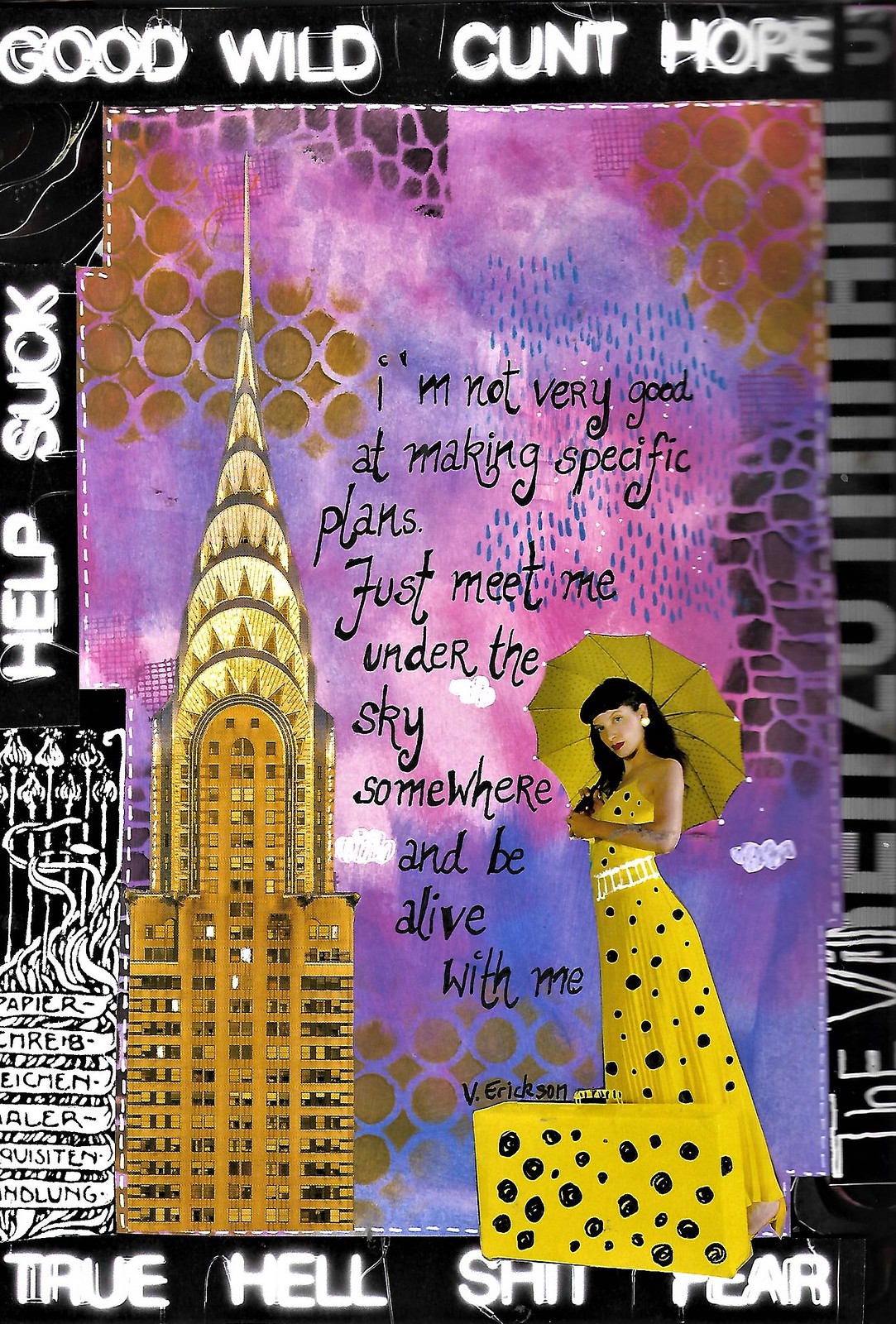The image showcases a rectangular piece of artwork, likely cropped from a web page, with a vibrant and multi-colored background featuring splashes of blue, purple, orange, red, and black. Prominently displayed in black script is the quote, "I'm not very good at making specific plans. Just meet me under the sky somewhere and be alive with me," attributed to V. Erikson. On the right side of the image, there is an artistic depiction of a woman with black hair, dressed in a sleeveless yellow tank top dress with black spots, holding a matching yellow umbrella. In front of her is a yellow suitcase with black dots. Beside this image, on the left, stands a tall, possibly iconic, brown building with a pointed top. The background along the edges of the artwork is black with white text scattered across different sections. The text includes words like "Good, Wild, Hope" at the top, and "True, Fear" at the bottom, along with other partially obscured or blurred words.